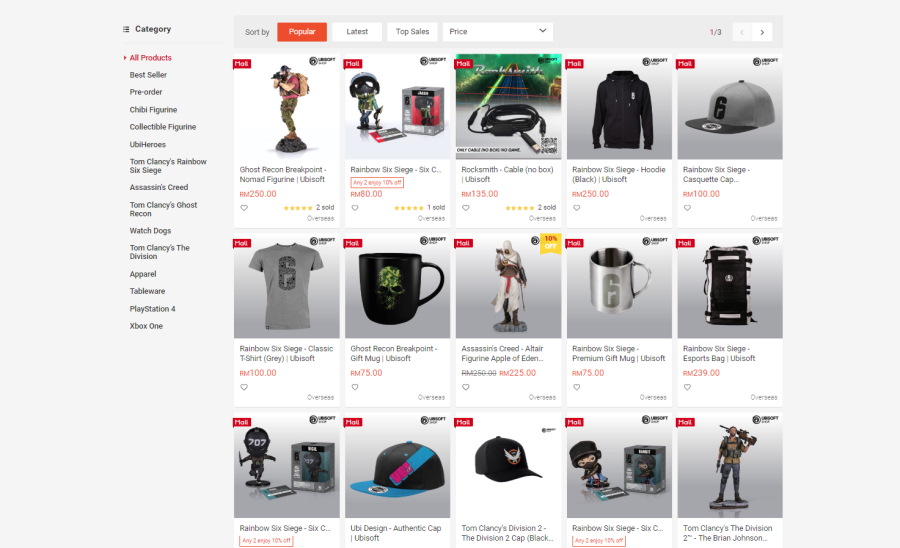The webpage image depicts an online store displaying various items, including models, cups, figurines, and hats, all set against a grey background. Each product is presented in a white box with pricing in red text and the item name in black text above it. The currency for the items is displayed in RM.

On the left side of the page, there is a mid-grey sidebar with black tabs for navigation. At the top of this sidebar, a category menu appears, with the 'Category' tab marked by three black lines on the left, indicating settings or filtering options. The 'All Products' category is highlighted in red with a red arrow, signifying it is currently selected, while the remaining categories are listed in black. The sidebar lists the following categories:

1. All Products
2. Best Seller
3. Pre-Order
4. Chibi Figures
5. Chibi Figurines
6. Collectible Figurines
7. UBI Heroes
8. Tom Clancy's Rainbow Six Siege
9. Assassin's Creed
10. Tom Clancy's Ghost Recon
11. Watch Dogs
12. Tom Clancy's The Division
13. Apparel
14. Tableware
15. PlayStation 4
16. Xbox One

At the top of the webpage, there is a dark grey banner featuring clickable buttons for sorting items. On the left side of this banner, black text reads 'Sort By.' One of the buttons is highlighted in red with white text indicating it is currently selected, and it reads 'Popular.' Next to it are two more buttons: a white one with black text labeled 'Latest' and another white button labeled 'Top Sales.' Additionally, there is a drop-down menu labeled 'Prices.'